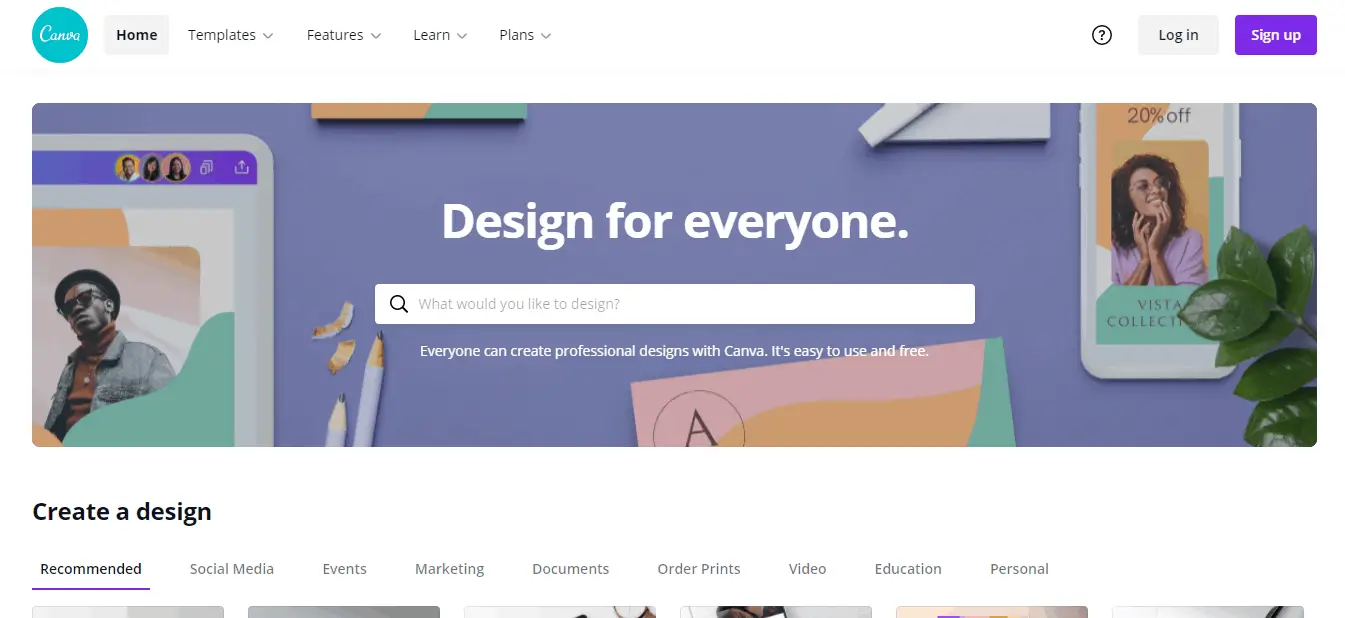Screenshot of the Canva Homepage

The screenshot captures the homepage of Canva, a design platform, showcasing its user-friendly interface with a primary focus on "Design for Everyone". At the top left corner, there's a blue circle logo with text "CAN" on it. A navigation menu adjacent to the logo includes categories like Home, Templates, Features, Learn, and Plans, with the Home button currently selected. On the top right, options for Help, Login, and Sign Up are displayed.

Below the navigation bar, a horizontally aligned section features a pastel-colored background in hues of purple, pink, orange, and green. A tablet on the left and a cell phone on the right display images created using Canva's design tools. Centered text reads "Design for Everyone" with a descriptive subtext below stating, "Anyone can create professional designs with Canva. It's easy to use and free."

Directly beneath this text is a white search box, followed by an invitation to "Create a Design". This is accompanied by a drop-down menu offering design categories such as Recommended, Social Media, Events, Marketing, Documents, Order Prints, Video, Education, and Personal.

The bottom portion of the screen hints at more design examples, though the images are partially obscured at the bottom edge of the screenshot. The overall background of the page is white, providing a clean and approachable aesthetic.